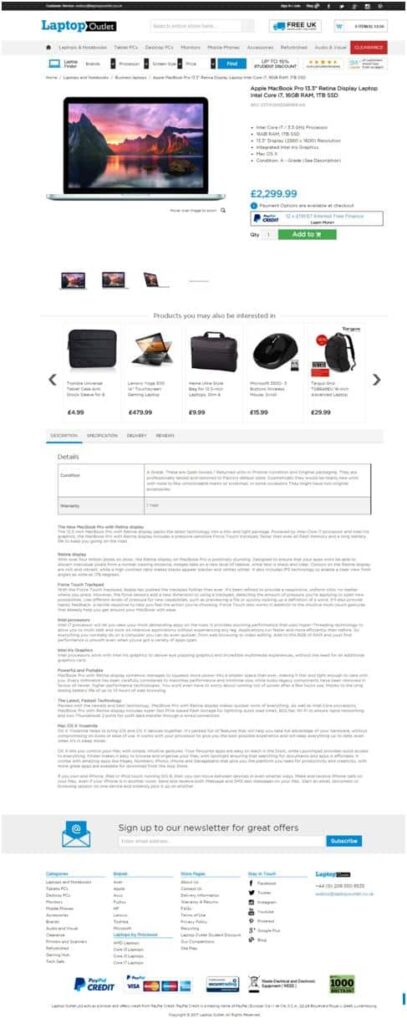Portrait-mode screenshot of a website:

The image opens with a black bar stretching across the top, featuring small and difficult-to-read white icons and text. The primary background of the website is white. In the top-left corner, bright blue letters spell out "Laptop," followed by an unreadable section of text in a black bar, hinting at an incomplete phrase like "Laptop something." A search bar is visible nearby, accompanied by a small ad that possibly mentions free shipping, indicated by a truck icon. Adjacent to this, another search bar is present.

Below this header, there are four small black squares with text, likely representing clickable categories. Centrally positioned is a large photograph of a sleek, elongated laptop. The laptop's display showcases a stunning image of a sunset over mountains reflected on a lake. To the right of the laptop, a price tag, potentially in pounds (£2,999.99), is listed. The detailed description of the laptop is minimal due to the small text size, but one can infer it contains specifications.

Directly beneath the laptop image, there are smaller thumbnail photos allowing users to view the laptop from different angles. A horizontal scrolling section featuring five different items—presumably laptop accessories like cases and mice—follows. Each item has a description and price listed below.

The lower half of the website contains extensive text, which is largely unreadable. There are four distinct categories available for selection, with the first category highlighted in blue, displaying its details. Below these categories, a light gray bar with a blue envelope icon encourages visitors to "Sign up to our newsletter for great offers," providing a field to enter an email address and a blue submit button next to it. The page concludes with dense, tiny text suspected to include locations, contact information, and payment method icons such as PayPal Credit, MasterCard, Visa, and possibly others like the Better Business Bureau.